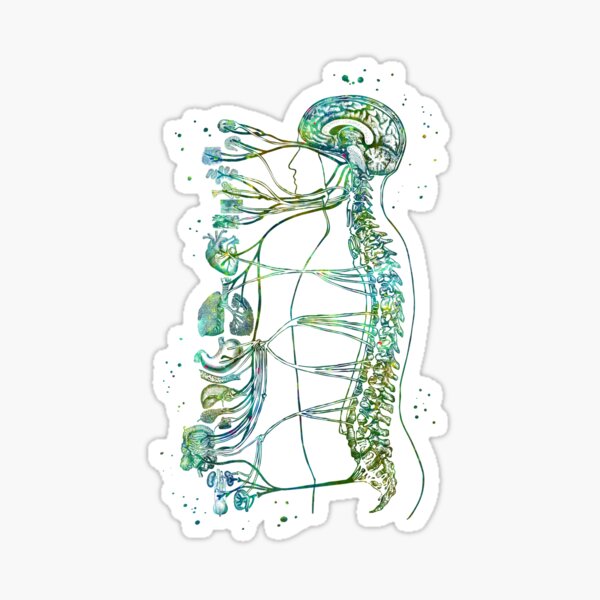This detailed sticker illustration features a whimsical, watercolor-like depiction of the human nervous system and associated organs, in various shades of green and blue, set against a white background. The image showcases the side profile of a male human torso, including the head down to the sacrum, outlined in black. Prominently, the brain and spinal column, illustrated in vibrant greens and blues, form the central focus on the right-hand side. Extending outward from the spine in intricate, vein-like tendrils, the diagram connects to several anatomically detailed organs positioned externally to the left, including the heart, lungs, liver, kidneys, stomach, intestines, and eyeballs. These organs and their connective nerves are depicted with the same green and blue colors, highlighting their association with the nervous system. Accentuating the vivid design, the outline of the entire sticker is irregularly shaped, dotted with coordinating color splashes, enhancing the artistic and biological essence of the illustration.